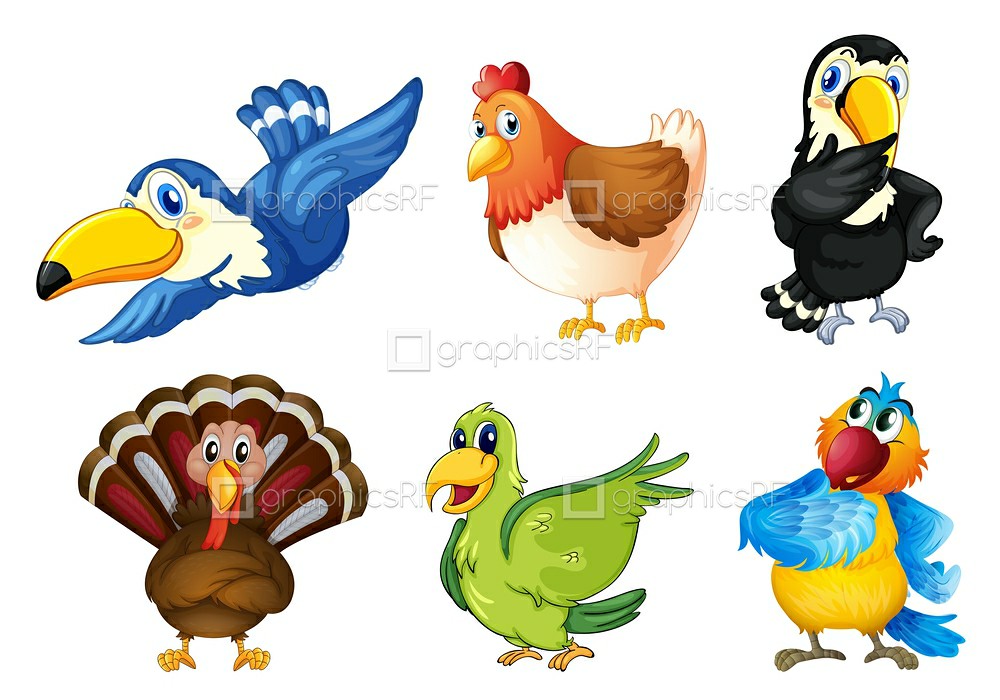The image features a collection of six cartoon birds, each representing different species and showcasing vibrant colors and varied poses. 

In the top left corner, there is a blue toucan with a prominent yellow beak. Adjacent to it, in the top middle, stands a uniquely colored chicken with an orange head, a red comb, blue wings, and a pale white body. The top right bird is another toucan, black in color, standing confidently with one wing positioned like a hand on its hip.

Moving to the bottom row, the bottom left bird is a brown turkey with red and gray feathers on its tail, wings folded in front of its chest. In the center bottom position, a green bird appears to be waving with a friendly demeanor. Finally, the bottom right features a bird with a yellow-orange body and head, complemented by blue wings and accents on its head, presenting a thoughtful expression.

The overall style of the birds suggests they are illustrations from a web page, depicted with a cartoonish charm.